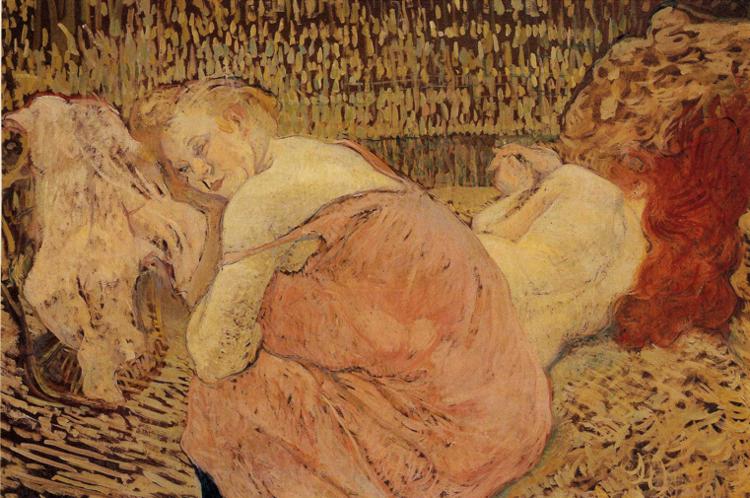The painting captures a detailed and intimate close-up of two women set against a contained, tan-brown background suggestive of an interior room. The central figure, an older, fuller-bodied woman with thin strands of blonde hair and small, squinty features, is clad in a voluminous, pinkish-orange gown that drapes over her stomach and legs. Her form is bent forward, and she twists her head back to meet the viewer's gaze with her pecky lips and squinted eyes, lending a sense of direct engagement. To her right, a red-haired woman lies on a bed, her back partially exposed and her arms extending towards the bed's edge. Her vibrant hair cascades upwards and downwards in flowing curls, creating dynamic movement within the frame. An ambiguous object, possibly clothing, rests on a brown rack to the far left, adding a touch of mystery to the scene. The painterly style balances touches of abstraction with realistic details, utilizing golden browns and darker hues to enrich the warm, intimate atmosphere.